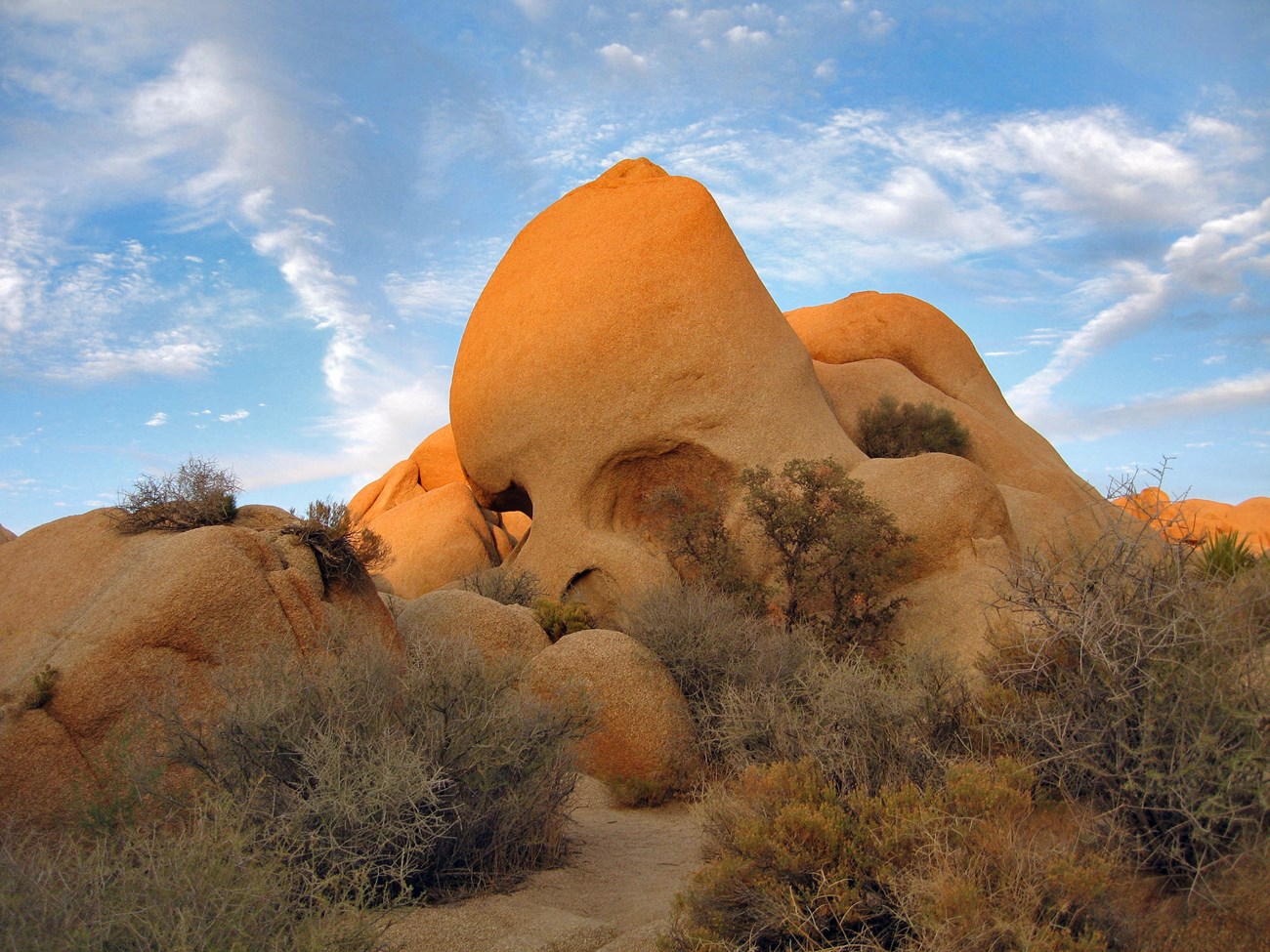In the image, there's a striking desert landscape during what appears to be the golden hours of either sunset or sunrise, with the golden hues suggesting it is more likely sunset. Dominating the scene is the iconic Skull Rock from Joshua Tree National Park, a large rock formation that strikingly resembles a human skull. Its rounded top and distinct cavities that mimic eye sockets, along with a small nose-like hole, create an eerie yet fascinating visage. The foreground is dotted with dry, thorny bushes and sparse, leafless brush, interspersed with patches of soft, sandy earth strewn with lighter-colored dirt. The boulders exhibit an orangish-brown tint, with the central one being the tallest and featuring a noticeable dent on its left side. The background showcases a series of similarly rugged, rounded rock formations, extending into a clear blue sky adorned with wispy white clouds. It's a quintessential desert scene, merging stark, rugged beauty with the ethereal light of dusk.